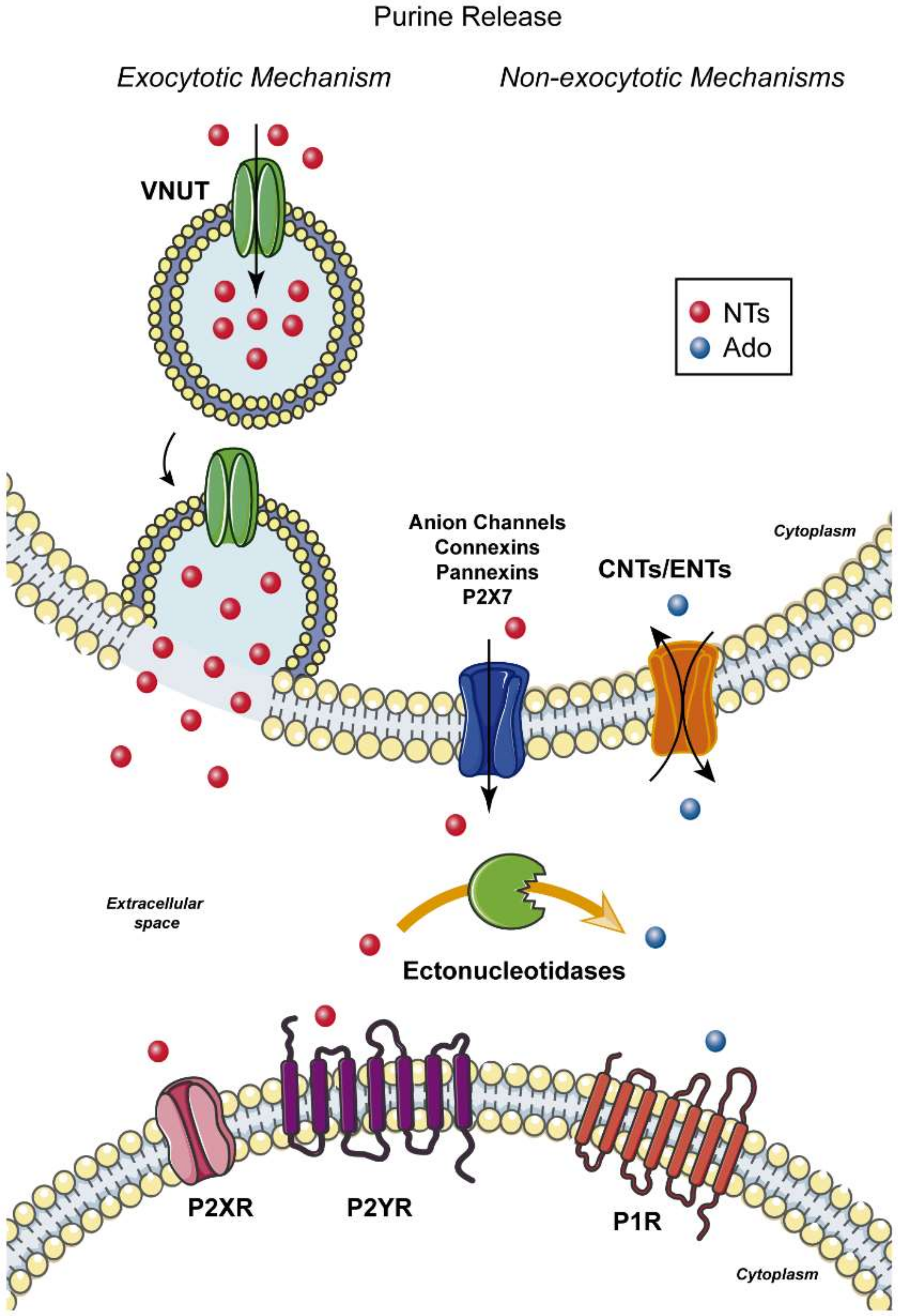The image is a detailed scientific diagram likely from a biology textbook, illustrating purine release mechanisms. At the top, it prominently states "Purine Release." Below this title, two mechanisms are specified: "Exocytotic Mechanism" and "Non-exocytotic Mechanisms." On the right, there is a square featuring a red dot representing NTs (neurotransmitters) and a blue dot representing ADO (adenosine).

The diagram includes several labeled sections and graphical illustrations. One diagram shows red dots (NTs) amassed within a circle, symbolizing vesicular packaging. Adjacent illustrations depict these red dots being released, suggesting an exocytosis process where vesicles fuse with the cell membrane to release their contents into the extracellular space. The term "Exocytotic Mechanism" aligns with this depiction.

Another part of the diagram illustrates non-exocytotic mechanisms, with blue elements labeled as anion channels and orange structures marked as CNTs and ENTs (concentrative and equilibrative nucleoside transporters, respectively). The cytoplasm and extracellular space are also labeled, with "Ectonucleotidases" indicating enzymes in the extracellular space that metabolize nucleotides.

Furthermore, the cytoplasmic section includes pink shapes marked as P2XR (P2X receptors) and purple shapes marked as P2YR (P2Y receptors), both involved in purinergic signaling. Adjacent are orange cylinders labeled P1R (P1 receptors), all interconnected with various colored lines depicting complex receptor interactions and pathways.

Overall, this comprehensive image provides an in-depth look at the cellular mechanisms of purine release, encompassing both vesicular and transporter-mediated processes, and highlighting the roles of various receptors and channels involved in these biochemical pathways.